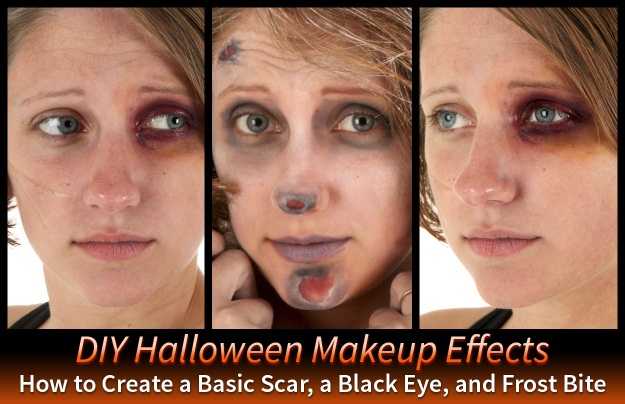The image showcases a step-by-step guide to creating DIY Halloween makeup effects, featuring three photos of the same woman against a black background with a gradient transitioning to a brownish-red at the bottom. At the very bottom in white text, it reads: "DIY Halloween Makeup Effects: How to Create a Basic Scar, a Black Eye, and Frostbite." The title is displayed in a gradient of letters fading from yellow to orange. The leftmost photo depicts the woman with dark makeup around her right eye to simulate a black eye, and she is looking to the right. The middle photo shows her facing the camera with detailed makeup imitating frostbite wounds on her upper right forehead, nose, and chin, with a mix of bluish-gray and reddish tones to enhance the effect. The rightmost photo again features the black eye makeup, but this time her head is turned to the left. The overall presentation serves as a visual tutorial on creating realistic Halloween makeup effects.